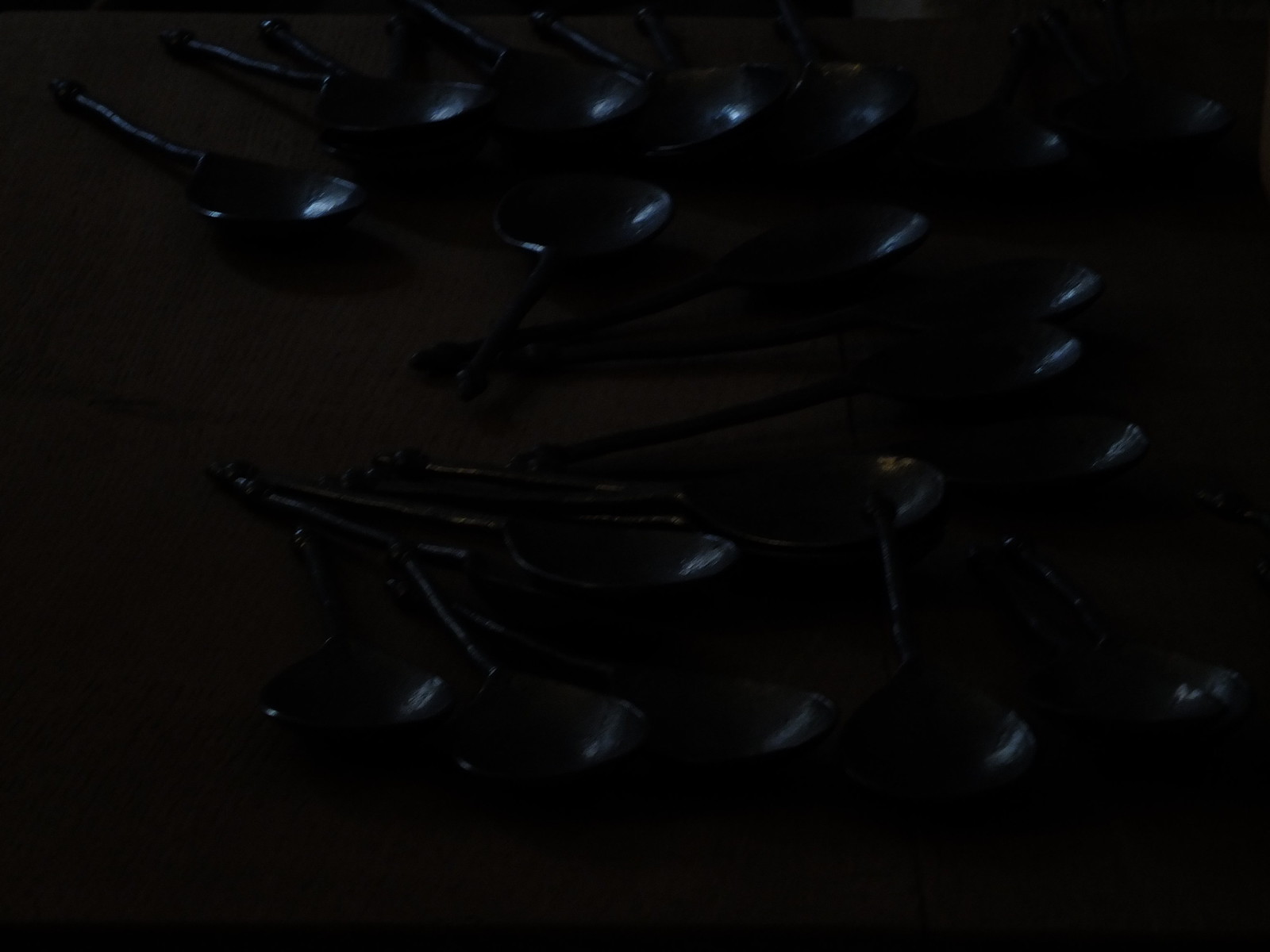The image depicts a very dark scene with a completely black background, likely representing a dark brown or black table surface. Scattered across this surface are numerous metal spoons, their precise color difficult to determine due to the low light—potentially silver, copper, or gold. The spoons possess unique circular handles, some of which appear to have a bolt-like protrusion. There are elongated tails or glints of light on the spoons, suggesting they might be moving or reflecting light. Positioned in varying orientations, the spoons seem loosely arranged, with some forming distinct rows or clusters, adding a sense of organized randomness. Notably, some spoons seem aligned from the top right corner to the bottom left, accentuating a floating illusion within the dark setting. The faint white lines and light reflections on the spoons add a subtle sparkle, breaking the otherwise pervasive darkness and providing just enough detail to discern their metallic sheen.